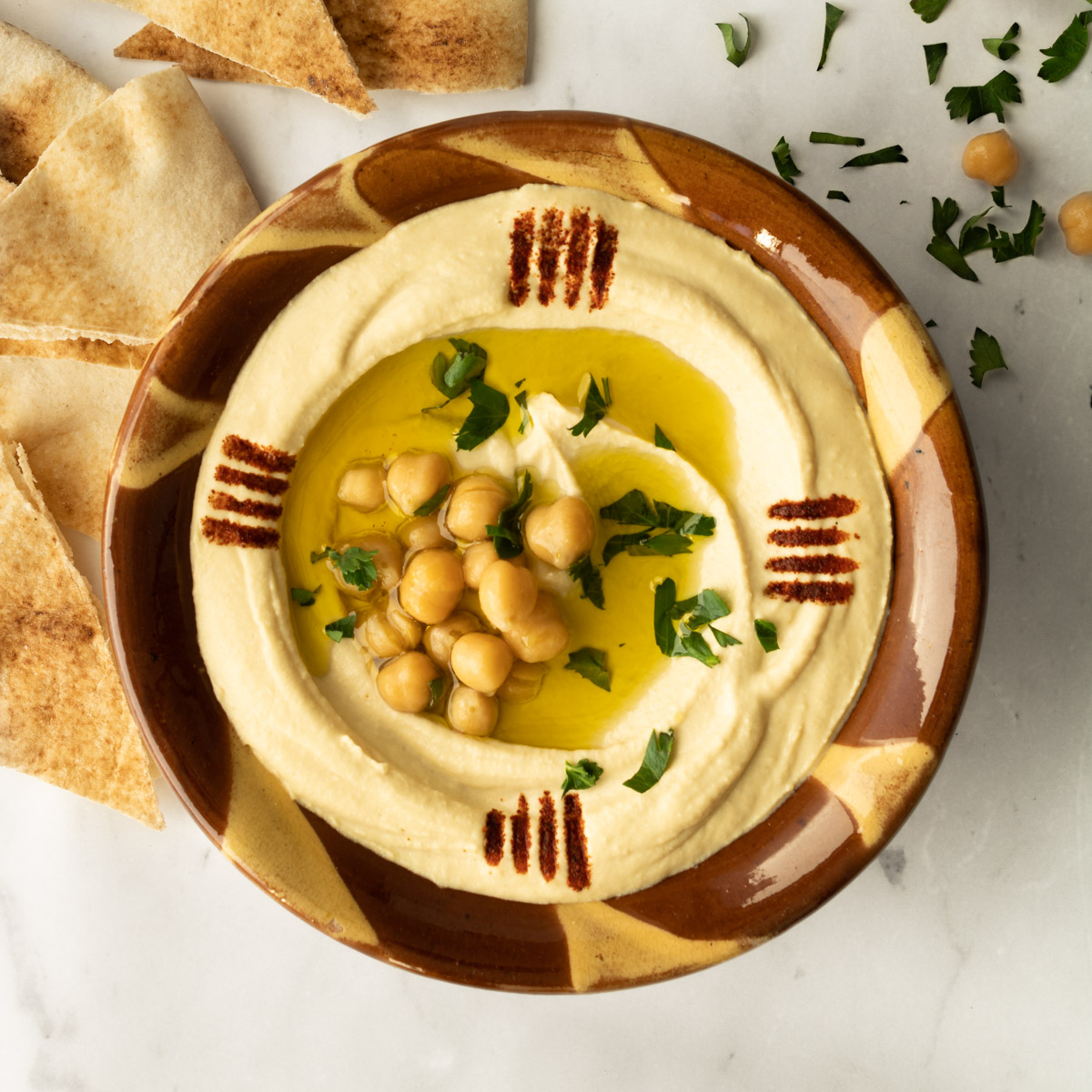This overhead shot captures a beautifully plated dish of hummus set on a white marble table. The hummus is served in a circular, glossy brown ceramic bowl adorned with light tan striations. To the left of the bowl, a scatter of crispy pita chips lies invitingly. The smooth, creamy hummus is artfully presented with four lines of paprika, creating a decorative touch at the north, south, east, and west positions. The center of the hummus features a well of golden olive oil, garnished with whole, unpureed garbanzo beans and finely chopped cilantro. Around the bowl, a few stray garbanzo beans and sprigs of cilantro add a casual touch to this elegant and inviting dish.